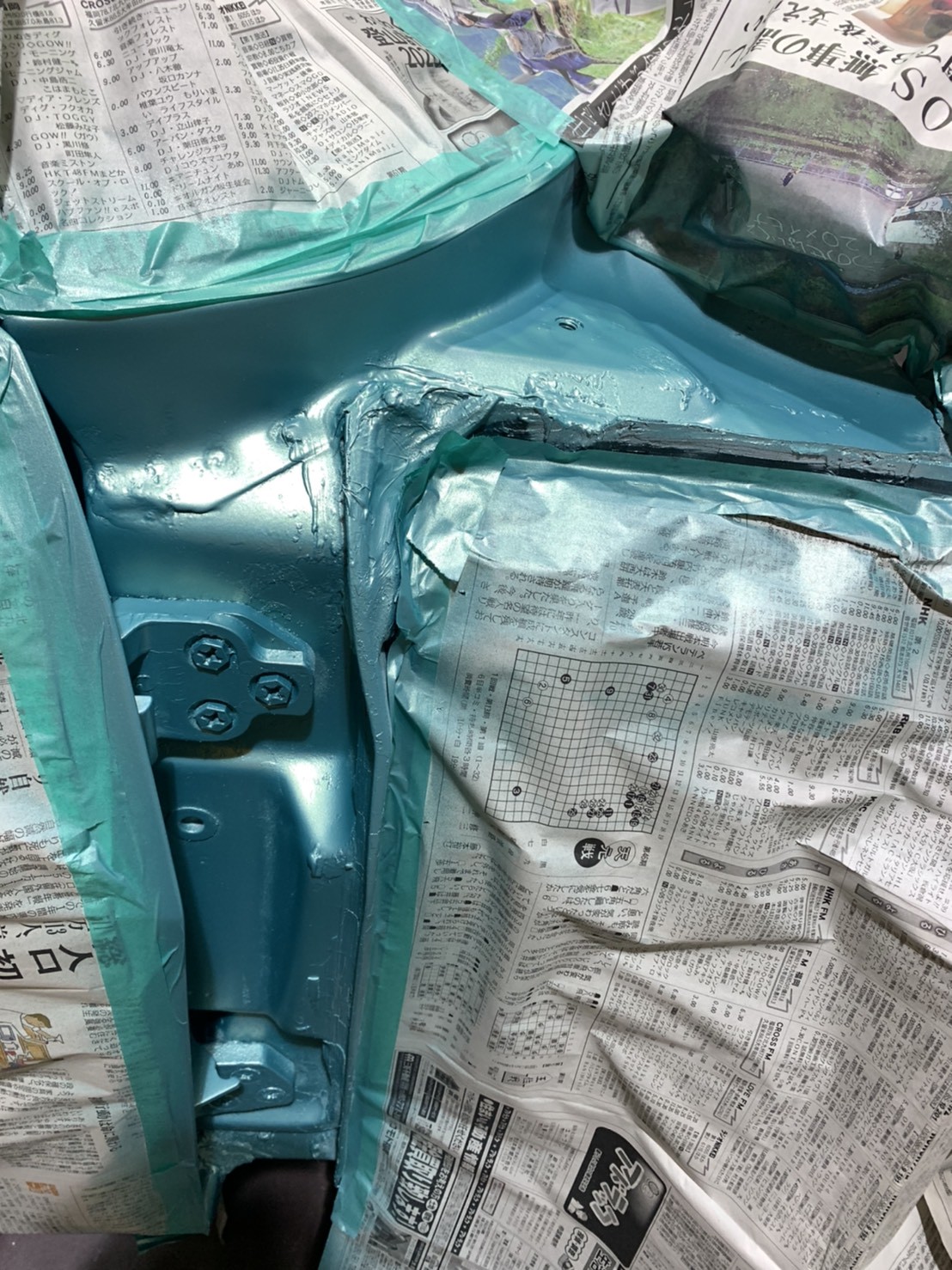This color photograph features a close-up of what appears to be a metallic object, likely a car or a machine, being spray-painted in a metallic aqua blue color. The object is covered partially in squares of newspaper that have been taped on meticulously with duct tape to presumably protect certain sections from the spray paint. The newspaper edges and some parts of the tape show signs of the same blue paint, suggesting it was applied after the coverings were set in place. The newspapers, displaying a mix of what looks like a crossword puzzle, classified ads, and Asian language text, are light gray with darker gray prints. The photograph offers an intimate glimpse into the process, highlighting the complexities of spray-painting with visible drips of paint and careful masking. No people are present in the image, and the tight framing makes it difficult to discern the complete context of the scene.